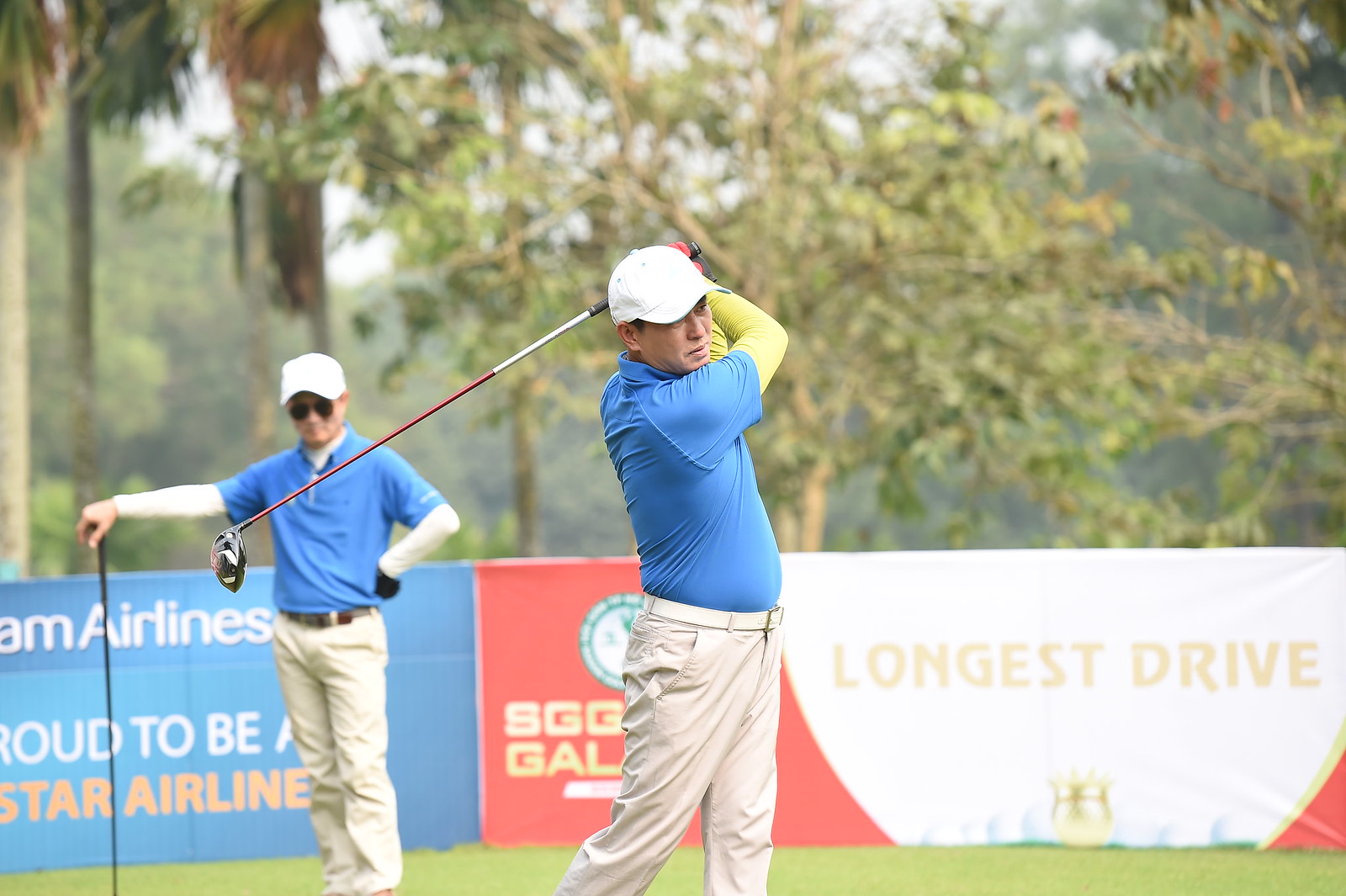This is an image of two men on a golf course, captured with detailed focus on the foreground and background elements. The man in the center of the image has just completed a swing, with his golf club extended over his shoulder. He is dressed in a blue short-sleeved collared shirt with a neon green long-sleeve undershirt, khaki pants, a white belt, and a white baseball cap. He’s also wearing bright red gloves. Just behind him to the left stands another man, who is similarly dressed in a blue short-sleeved shirt, a white long-sleeved undershirt, khaki pants, a brown belt, and a white baseball cap, although this man also sports sunglasses and is casually leaning on his golf club, which stands upright. Both men are positioned on a vibrant green tee box. In the background, there are advertising banners: one from an airline that reads “Proud to be a 5-star airline” and another that mentions the “Longest Drive” competition. Additionally, the banner for “SGG Galaxy” is partially visible. Behind the banners, lush green trees are visible under a slightly overcast sky, adding depth to the setting.